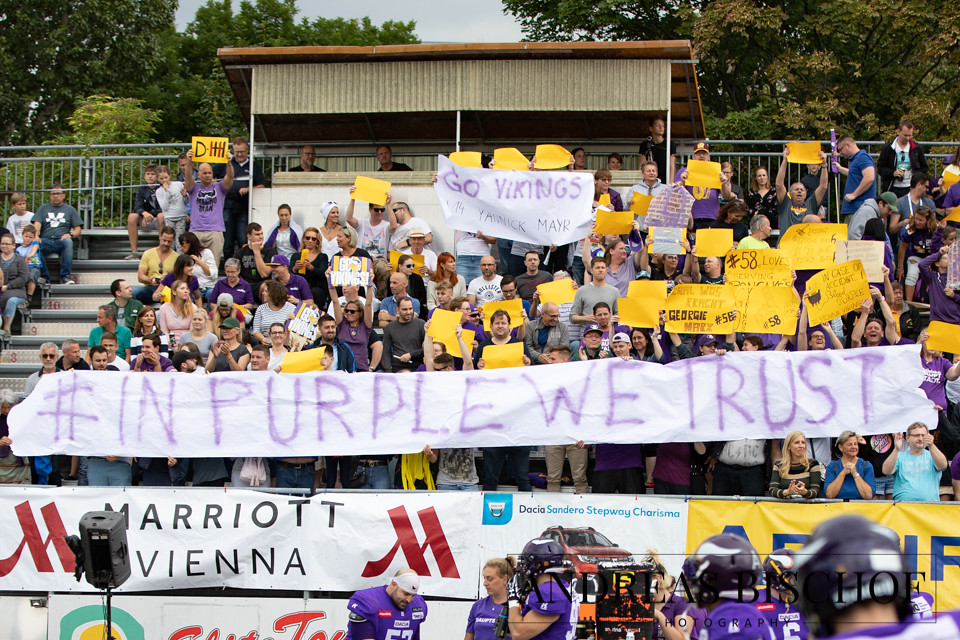The image captures a lively daytime football event, likely a high school game. In the foreground, football players donning blue uniforms with the iconic Minnesota Vikings' purple helmets and white Viking horn logos are visible. The stands are filled with cheering spectators, many of whom are holding vibrant yellow signs primarily featuring the number "58" and various other messages, including references to "George Marks #56." Prominently displayed at the front of the crowd is a large white banner with the phrase "In Purple We Trust" written in bold purple letters, supported by approximately 20 people. Above it, a smaller sign reads "Go Vikings." The announcer’s booth, an open wooden structure with a roof, is seen atop the stands, housing commentators. Surrounding this scene are lush, tall green trees, and banners with sponsorships like "Marriott Vienna" are displayed along a barrier. Additionally, there's a woman in a blue shirt among the spectators, indicating diverse attendee attire and involvement. The overall atmosphere is energetic, with a palpable sense of community and support for the local team.